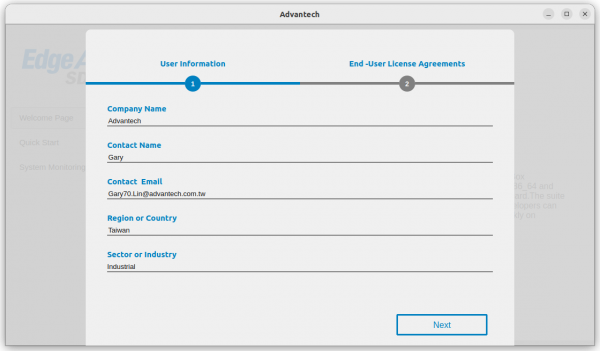The image depicts a pop-up window from a website called AdvanTech. At the top of the screen, the name "AdvanTech" is prominently displayed on the web bar, accompanied by the typical minimize, maximize, and close buttons in the top right corner.

Beneath this header bar, there is a pop-up window with a faint gray background, divided into two stages: "User Information" and "End-User License Agreements." The "User Information" tab is currently highlighted.

Within the "User Information" section, there are five input fields organized in a vertical layout:

1. **Company Name:** This field is pre-filled with "AdvanTech."
2. **Contact Name:** This field is pre-filled with "Gary."
3. **Contact Email:** This field is pre-filled with "Gary70Lin@AdvanTech.com.tw."
4. **Region or Country:** This field is pre-filled with "Taiwan."
5. **Sector or Industry:** This field is pre-filled with "Industrial."

Each section header is in a bright blue font, while the input fields themselves are dark gray. At the bottom right of the pop-up, there is a blue, clickable box outlined with white, bearing the word "Next" in the same blue hue as the outline.